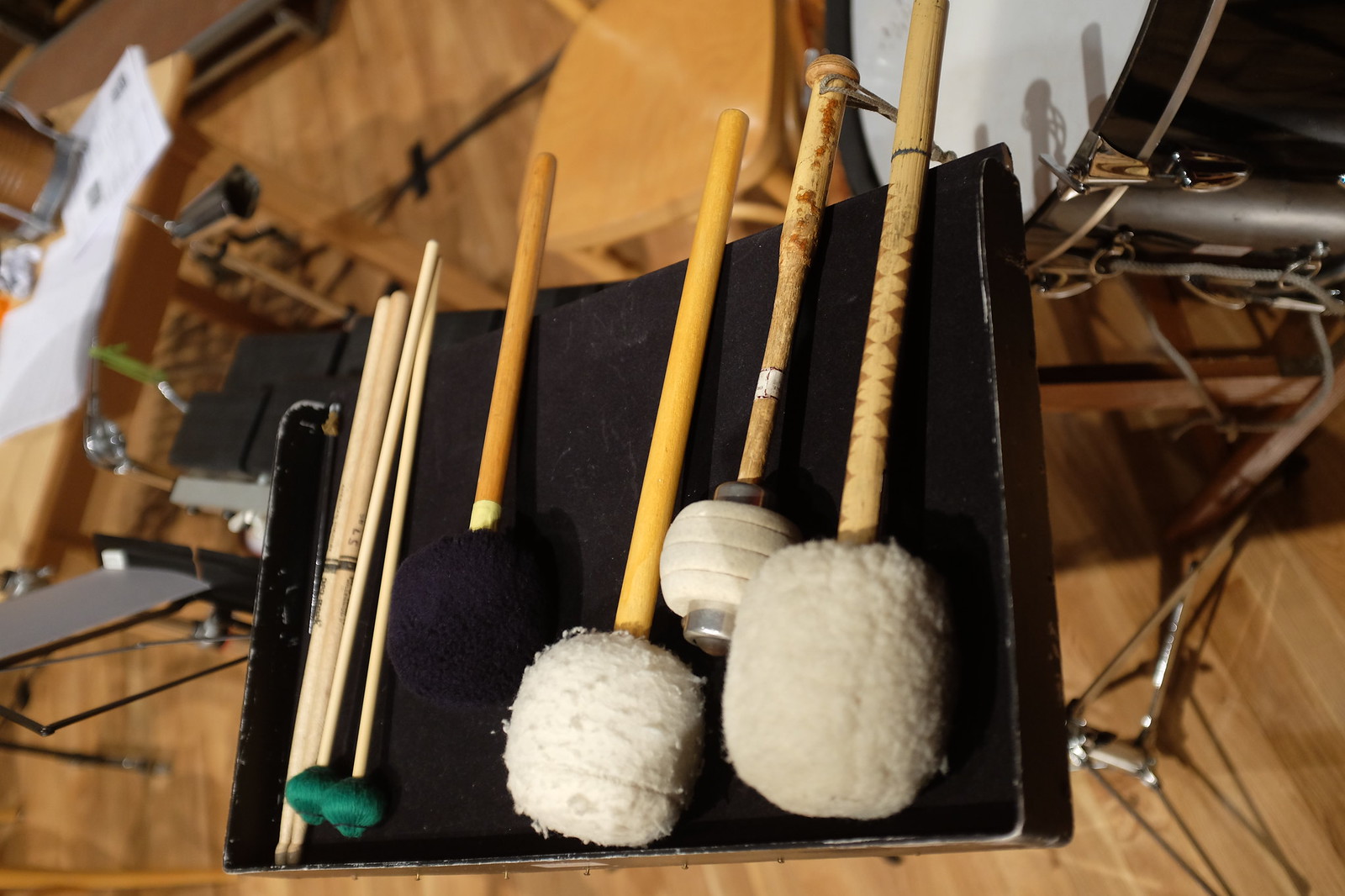The photograph, taken indoors from an overhead angle, features a medium color wooden desk positioned on a light brown tan wooden floor. Resting on the desk is an open black tray containing various percussion tools. Prominently displayed are several drumsticks and mallets, all equipped with wooden handles. The mallets are distinguished by their varied tips; three feature white wool, one has black wool, while others have green yarn tips. Additionally, there is a larger mallet with a brown handle and a woolen fabric, plus another with metallic ends. Adjacent to the tray sits metal equipment, partly obscured, and a round wooden stool positioned on the floor further emphasizes the organized yet intricate display of the percussion instruments. In the upper right section of the image, the lower portion of a drum with a black frame is visible, tying together the musical context of the scene.